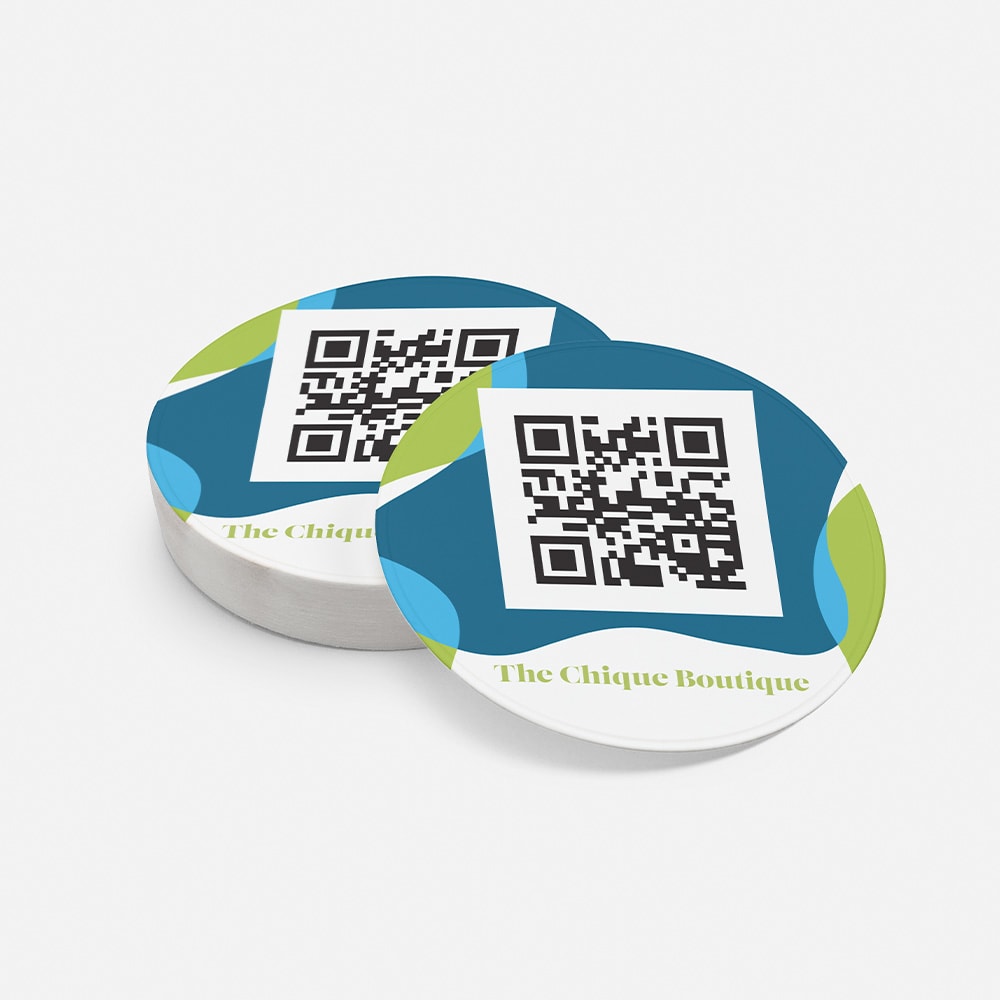This promotional image features a neatly stacked set of circular drink coasters designed to protect surfaces from drink condensation. The coasters showcase eye-catching abstract patterns, including dark blue, green, and white blobs. Prominently, each coaster displays a large, square-shaped QR code composed of black pixelated lines, situated at the center. Below the QR code, in green text, is the brand name "The Cheek Boutique.” The coasters are against a light gray background, with one coaster slightly slid off to the left, casting a gentle shadow and adding a sense of dimension. The photograph emphasizes the uniformity and intricate design of the coasters, underlying the promotional intent for The Cheek Boutique's product line.